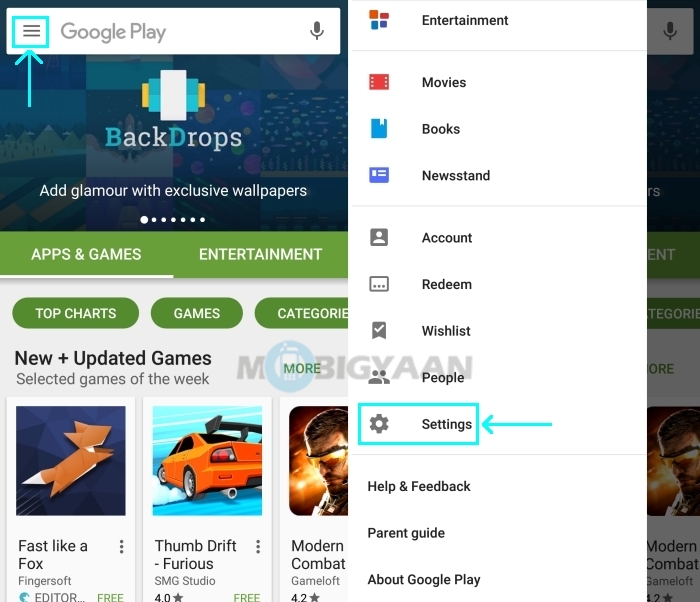This screen capture showcases the Google Play Store page, highlighting an exclusive selection of wallpapers under the heading "Backdrops: Add Glamour with Exclusive Wallpapers." The backdrop is vividly designed with a combination of turquoise, yellow, and white colors. The page is set to the 'Apps & Games' tab, as indicated by the highlighted section. 

Beneath the main heading, there's a featured segment titled "New and Updated Games," showcasing a variety of recently updated games. The first game listed is "Fast like a Fox" by Fingersoft, labeled as an editor's pick. Accompanying it is a colorful graphic suggesting dynamic gameplay. Next to it is "Thumb Drift: Furious Racing" that features an image of a drifting car, conveying high-speed action with squealing tires and flying dust. The next game's title is partially visible but identifiable as "Modern Combat" by Gameloft, hinting at an intense, action-packed experience. This detailed visual offers a glimpse into the latest trends and updates in mobile gaming available on the Google Play Store.